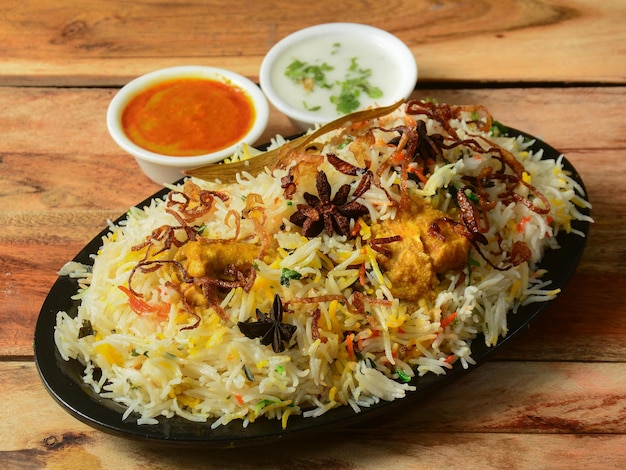This color photograph captures an up-close image of a dish resting on a wooden table. The main focus is a long, black, oval plate heaped with a mix of long-grain white and yellow rice. Atop the rice, there is a colorful array of ingredients including pieces of fried chicken, caramelized onions, and various garnishes in shades of red, orange, and green. There are also flecks of a pale orange-pink seasoning sprinkled throughout. Draped across the dish are strands of a light brown vegetable, possibly resembling thin ribbons or a spoon in shape. Adjacent to the plate, there are two small white cups; the one on the left contains a yellowish-orange sauce, while the one on the right holds a white sauce garnished with green flecks. The image is taken at a slight angle from above, emphasizing the vibrant and diverse elements of the meal against the rustic wooden background.